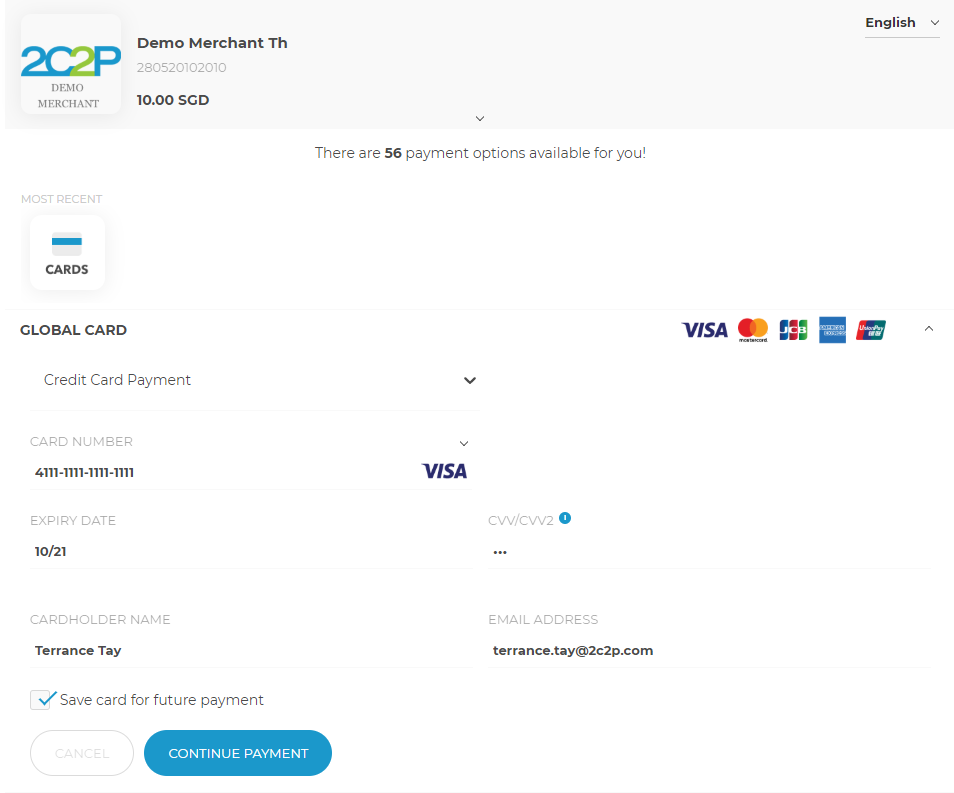A screenshot of a desktop application, likely a demonstration of a credit card payment processing system from "2C2P Demo Merchant," is displayed. The interface is clean with a primarily white background and soft off-white, slightly shaded input boxes. The top of the screen features the logo "2C2P Demo Merchant" followed by a displayed amount of $10 SGD, indicating the transaction value.

In the main body of the screenshot, various fields are available for input, with sections for entering the credit card number, cardholder's name, and the card type, which has been selected as Visa. The card number and cardholder's name fields are already populated. A checkbox option to save the card details for future transactions is also visible.

Below the input fields, there is a space to enter an email address, which in this instance is Terence Tay's, matching the company's email domain. Two prominent buttons labeled "Continue Payment" and "Cancel" are present for proceeding with or halting the transaction.

On the right-hand side of the interface, logos representing various card types are neatly arranged. The overall design is user-friendly, with drop-down menus, clickable tick boxes, and buttons to facilitate the filling of required details for processing credit card payments. This screenshot showcases a straightforward and efficient payment processing demonstration.